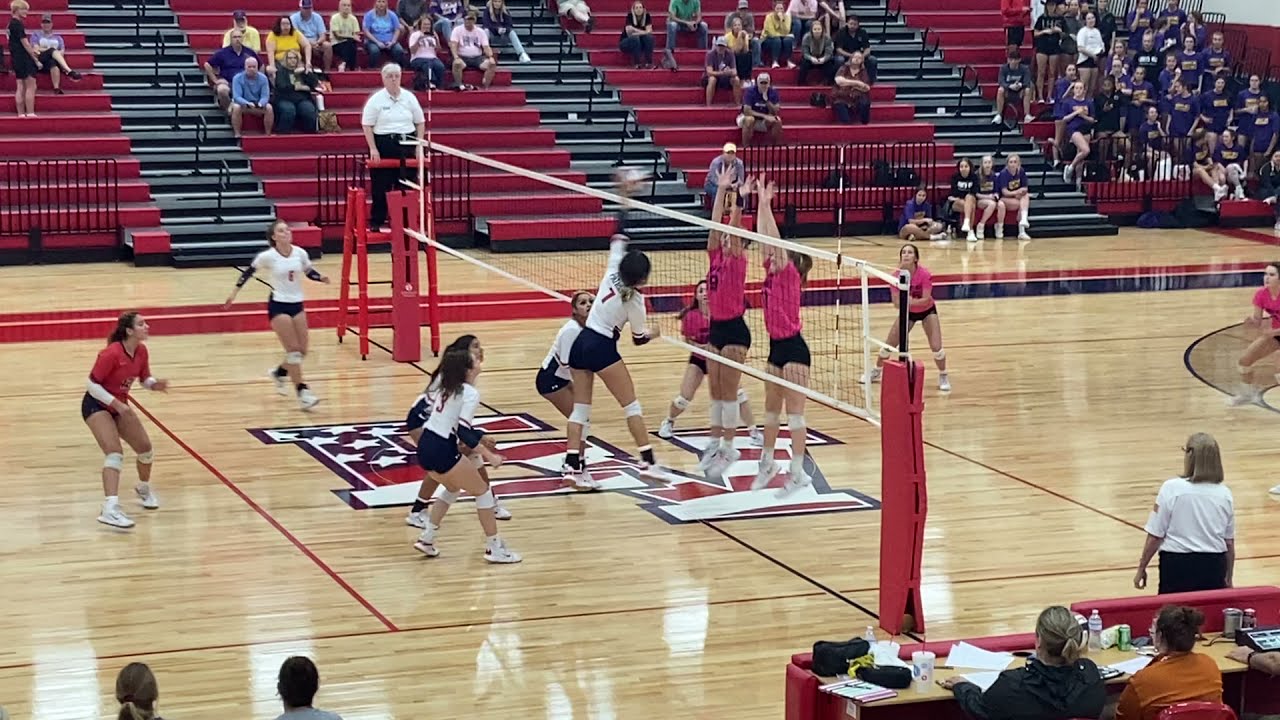This vibrant image captures the high-energy atmosphere of an indoor volleyball game held in a sports arena with red bleachers filled with spectators. The focal point is the wooden, shiny floor decorated with a central logo featuring an 'EV' stylized with American flag elements, with red, white, and blue lines as well as white stars. The volleyball court, which also doubles as a basketball court evidenced by the visible three-point line, is divided by a net. 

Two teams are in mid-action: the team on the left, wearing white shirts with blue shorts, and the team on the right, dressed in pink shirts with black shorts. A player from the team on the left is captured spiking the ball over the net, while two players from the opposing team leap to block it. The referees, clad in white shirts and black pants, rigorously oversee the match, one positioned atop a referee stand.

In addition to the engaged crowd in the bleachers, there’s another team seated in the top right stands, indicating that this is likely part of a larger tournament. The scorer's table is also in view, adding to the organized chaos of the live event. The scene is bathed in a palette of colors, including light brown, white, red, black, blue, orange, yellow, and tan, highlighting the dynamic and spirited environment of the game.